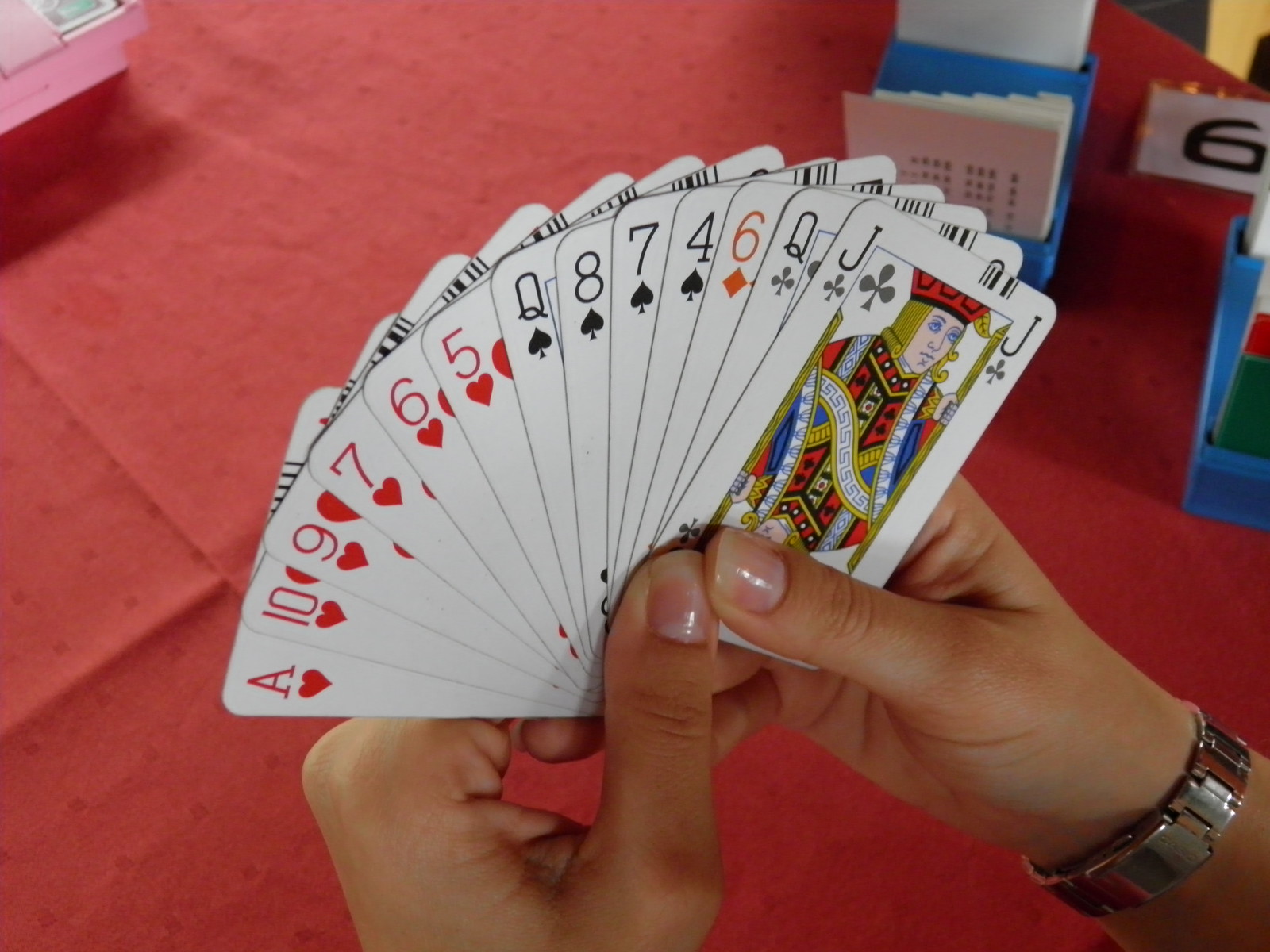A person with light skin is prominently featured in the foreground, holding a fan of cards with both hands. They are wearing a silver watch on their right wrist, and their shiny nails are unadorned with any colored polish. The cards, shown in perfect clarity, are arranged in a specific order: ace of hearts, 10 of hearts, 9 of hearts, 7 of hearts, 6 of hearts, 5 of hearts, queen of spades, 8 of spades, 7 of spades, 4 of spades, 6 of diamonds, queen of clubs, and jack of clubs. The background, intentionally blurred to emphasize the person and the cards, reveals a table draped with a red tablecloth, which has visible folds. In the corner of the image, a pink object is partially cut off. Two blue containers, seemingly used to hold more cards, are placed further back on the table. A laminated piece of plastic displaying either the number six or nine (depending on orientation) is also visible. Light illuminates the table and casts shadows on both the containers and the person's hands, adding depth to the composition.